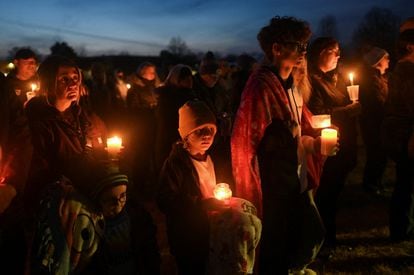In the dim twilight, a poignant scene unfolds in this image capturing a somber vigil. Central to the image is a child kneeling, softly illuminated by the glow of the candle they clasp in their hands. The child wears a hat, a white shirt, and a dark jacket, embodying the earnestness of the moment. To the child's right, a taller figure also kneels, draped in a red jacket or shawl, their candle casting elongated shadows. Further to the right, another individual holds a candle, standing slightly apart from a man in the far back, identifiable by his hat in the top-right corner of the image. On the left side of the child, a person with longish blonde hair cascading to their neck kneels, candlelight flickering over their contemplative face. Behind them, another man holds a candle, his form faint against the last vestiges of daylight in the pale blue sky. The gathering, composed of people of various ages bundled in hats, coats, and scarves, suggests cold weather. Though the image quality is poor, and individual faces are indistinct, the collective posture and illuminated candles indicate a communal act of remembrance or prayer, set against the encroaching darkness.